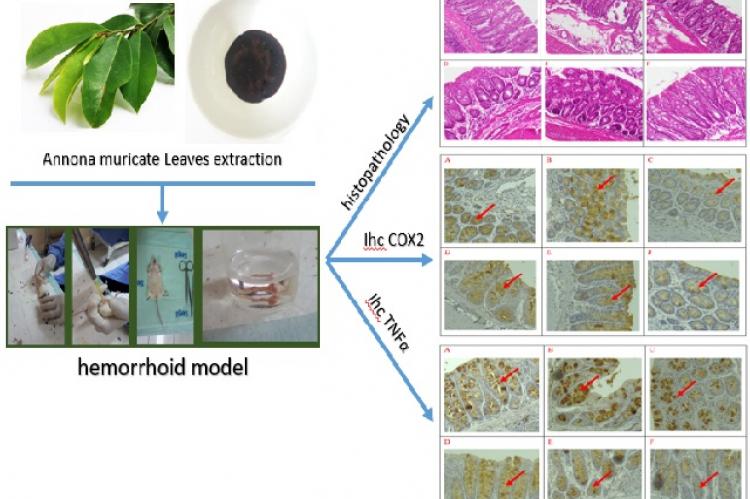The image is a detailed scientific diagram on a white background. In the upper left corner, there's a small branch with green leaves, labeled "Anona muricata leaves extraction." Below this, there's an illustration of an experiment seemingly involving a rodent eye or possibly the extraction of a substance. This section is followed by the label "hemorrhoid model." A blue arrow points downward from this section. On the right side of the diagram, there are three blue arrows each pointing to different clusters of six microscopic images, totaling 18 images. The upper arrow points to images labeled "Histopathology," which are purplish in color. The middle arrow, labeled "IHCCOX2," points to grayish-tan images with small red arrows. The bottom arrow points downward to images labeled "LHC TNFA," similarly colored to the middle set. Each cluster of images appears to show cellular or tissue-level details, suggesting a focus on microscopic and histological analysis.